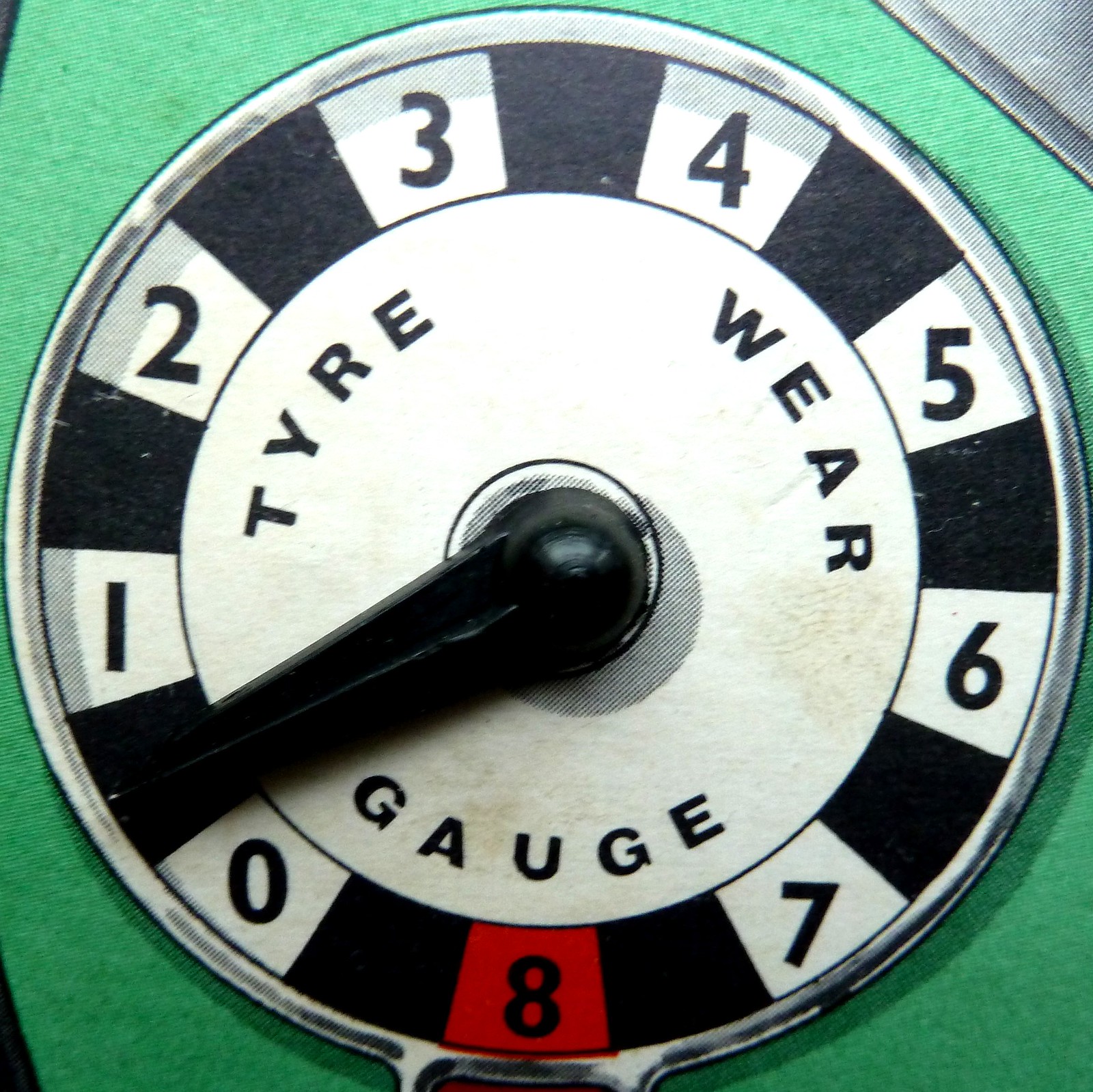The image features a tire wear gauge positioned against a light green background. The gauge is circular with a silver rim and occupies the majority of the image, centered prominently. The gauge is designed with alternating black and white checkered segments along the outer edge, each white segment containing black numbers ranging from 0 to 8, with the number 8 in red positioned at the bottom, indicating the highest level of wear. In the middle of the gauge, there is a white circle with the text "TIRE WEAR GAUGE" displayed in black letters, with "TIRE" on the top left, "WEAR" on the top right, and "GAUGE" at the bottom center. The black dial extends from the center towards the bottom left, pointing between the numbers 0 and 1.